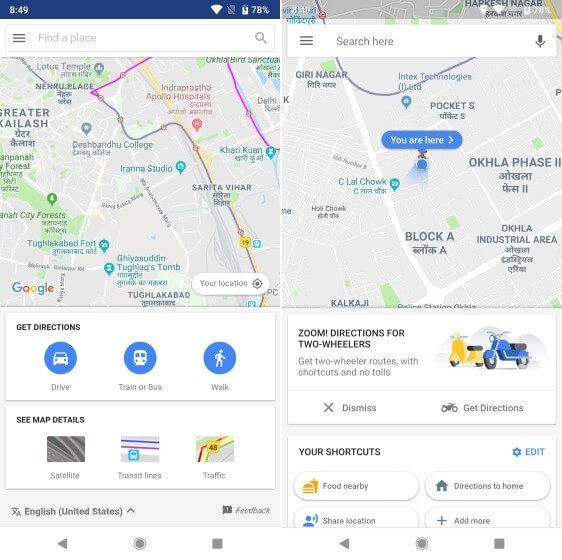Below is a detailed and cleaned-up caption for the image described:

---

**Side-by-Side Comparison of Mapping App Interfaces**

The image features two screenshots from a mapping application displayed side-by-side. Both screenshots display the time as 8:49, and the battery level is shown at 78%.

**Left Screenshot:**
- The top menu features a blue bar and a search field labeled "Find a place."
- A detailed map area is visible below the search bar, highlighting several notable locations:
  - Greater Kailash
  - Desh Bandhu College
  - Iranna Studio
  - Tughlaqabad
- Navigation options are available below the map, including "Get directions" with options for "Drive," "Train or Bus," and "Walk." 
- Users can also see additional map details such as "Satellite," "Transit lines," and "Traffic."
- The interface language is set to "English (United States)."

**Right Screenshot:**
- The top menu features a gray bar and a search field labeled "Search here."
- In the center of the map, a blue dot with the label "You are here" indicates the user's current location.
- Surrounding areas include:
  - Giri Nagar
  - Okhla Phase 2
  - Okhla Industrial Area
- Below the map, users can access "Zoom directions for two-wheelers," offering routes with shortcuts and no tolls.
- Options at the bottom include "Dismiss" or "Get directions," along with shortcuts for "Food nearby," "Directions to home," "Share location," and "Add more."

These detailed functionalities and layouts serve to guide users effectively through different navigation and location services, catering to various commuting needs and preferences.